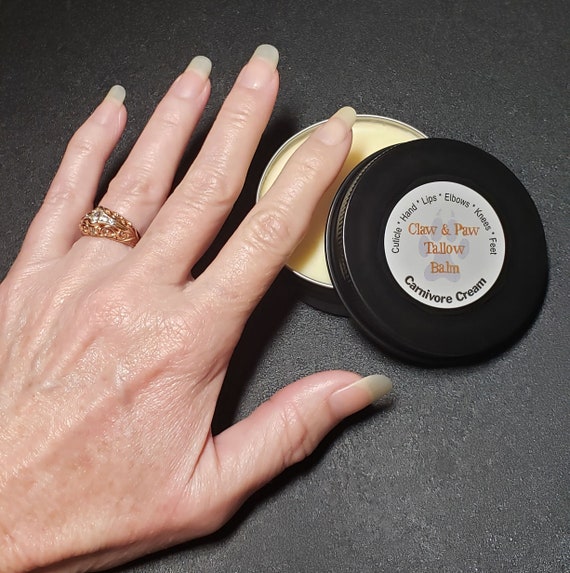This color photograph showcases a close-up view of a Caucasian woman's left hand resting on a pebbled gray tabletop surface. The woman appears to be middle-aged, possibly over 70, given the visible wrinkles on her pale skin. Her fingernails are long and glazed with a clear polish, and she wears a gold ring with a stone setting on her ring finger. Centered under her left index finger is an open black metal can containing a yellow, waxy substance, identified as Claw and Paw Tallow Balm. The lid of the can, also black, is partially resting on the container, adorned with a white circular label reading: "Claw and Paw Tallow Balm Carnivore Cream" and listing its uses for cuticles, hands, lips, elbows, knees, and feet. The image is brightly lit with natural lighting, enhancing the clarity and fine details of the scene.